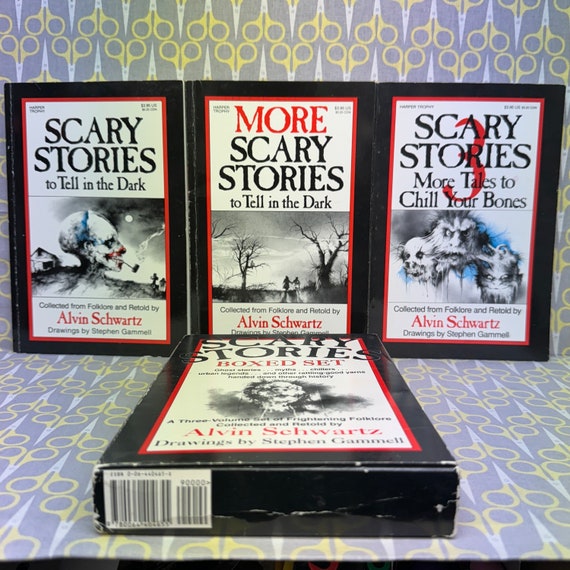The image features a set of four old and slightly worn books against a backdrop of stylized scissors with yellow handles and silver blades. The books are part of a series titled "Scary Stories" authored by Alvin Schwartz, with illustrations by Stephen Gammell. Three of the books are standing upright in the back, while a box labeled "Scary Stories Boxed Set" lies flat in the foreground. The upright books are black with white rectangles framed in red on their covers, featuring a mix of black and red text in a serif font. The titles and details of the standing books are:

1. "Scary Stories to Tell in the Dark" - The cover image shows a skull-like head emerging from the ground, smoking a pipe with gravestones and a moonlit night in the background.
2. "More Scary Stories to Tell in the Dark" - This cover features two people walking hand-in-hand through a stark, dusky landscape with two eerie bare trees.
3. "Scary Stories 3: More Tales to Chill Your Bones" - The cover depicts three monstrous faces, including what appears to be a pig-like creature, a werewolf, and a troll, each with distinct expressions.

The flat box in the foreground, which appears to hold the three standing books, reads "Scary Stories Boxed Set: A Three-Volume Set of Frightening Folklore" with similar text and illustration credits. The backdrop of the image is a light blue fabric with a repeating pattern of scissors, adding a quirky and slightly unsettling contrast to the eerie theme of the books.